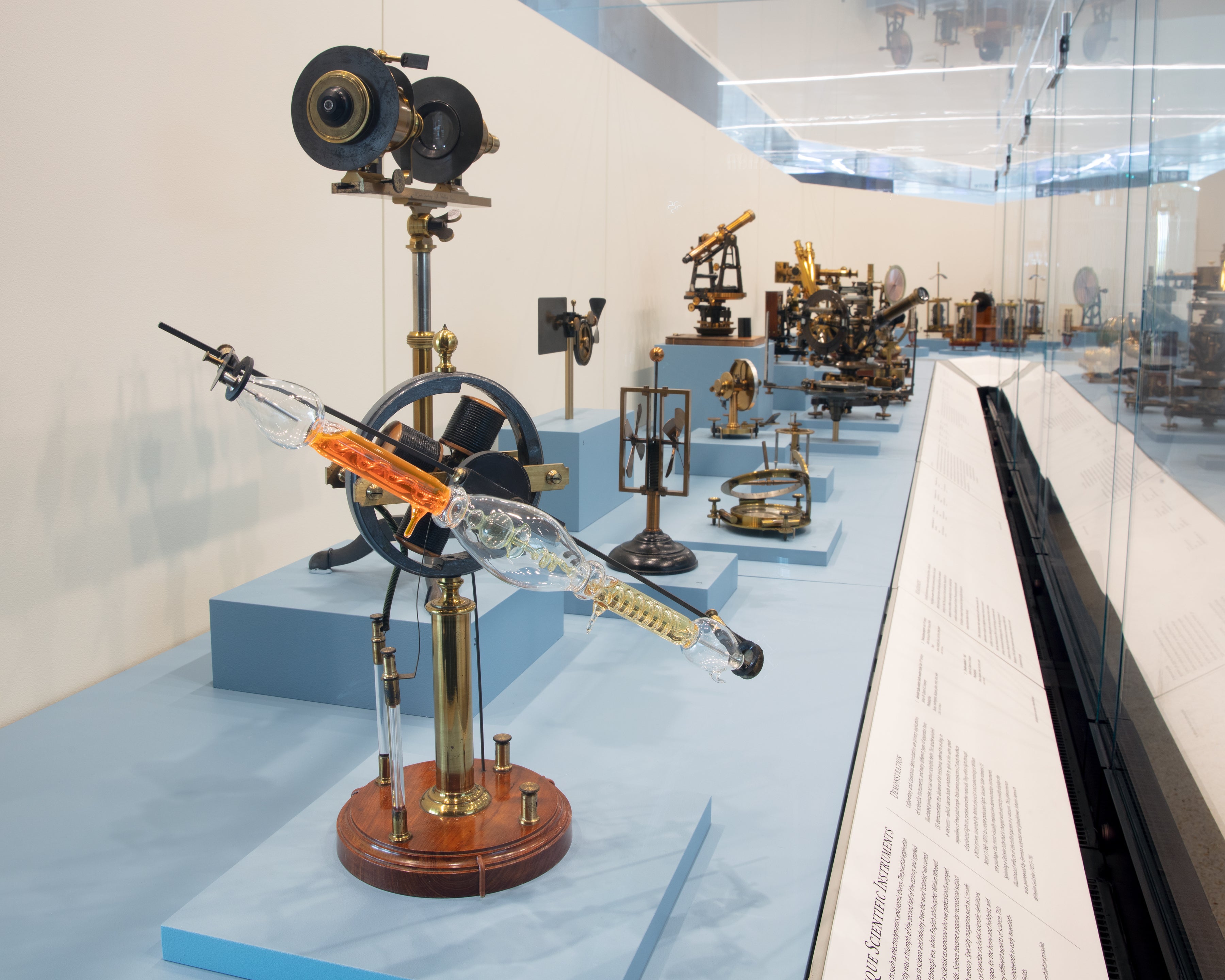The photograph depicts an indoor museum exhibition shelf with a blue base, showcasing a variety of historical scientific instruments. These instruments, primarily composed of metallic and glass components, include items that resemble telescopes. The majority of the metallic parts are golden, with some instruments featuring a brown, wooden-like base. On the right side of the shelf, there's a panel with text providing information about the displays, though the text is not legible from the viewing angle. The left side background wall is white, and the exhibit is encased by reflective glass panels on the right and above the shelf. Additionally, there are various blue square pedestals of different heights on which these instruments are placed. The general setup includes signs tilted towards viewers on the opposite side of the glass for better readability. The nearest instrument appears to be a noble gas light with a central bulb and connecting coils.